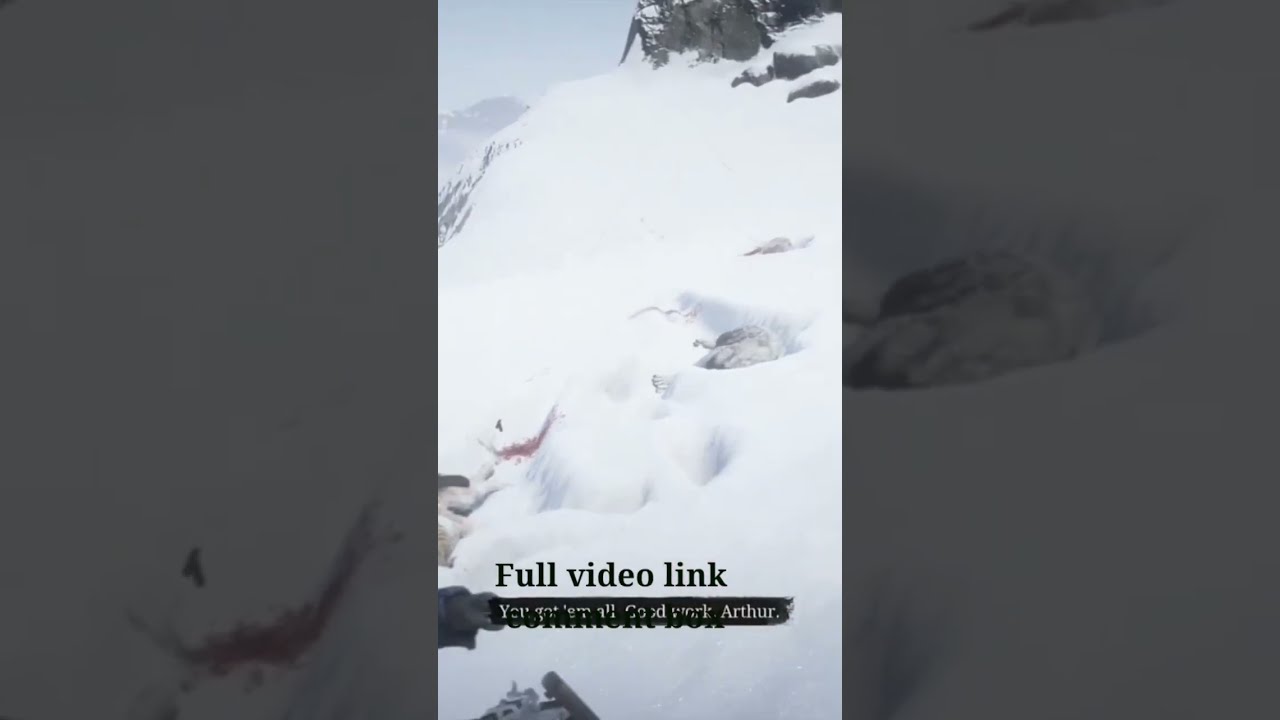The image consists of three panels, with the outer panels being dark, underexposed, and magnified sections of the brighter, normally lit central panel. The middle panel depicts a snowy mountain scene. Dominated by a mid-range mountain covered in fluffy, powdery snow, the terrain is jagged with rocks protruding through the snowy surface. The background suggests an overcast sky with possible sunlight, and the faint outlines of other mountains may be visible. The bottom left-hand corner of the central panel hints at a person, with what seems to be a foot or an arm partly visible. Overlayed on the scene, the bottom of the image contains black text stating "Full video link" followed by a black banner with white text reading "You'll get them all. Good work, Arthur," suggesting that the image could be a screenshot from a video game. Additional, smaller black text is present but not legible.